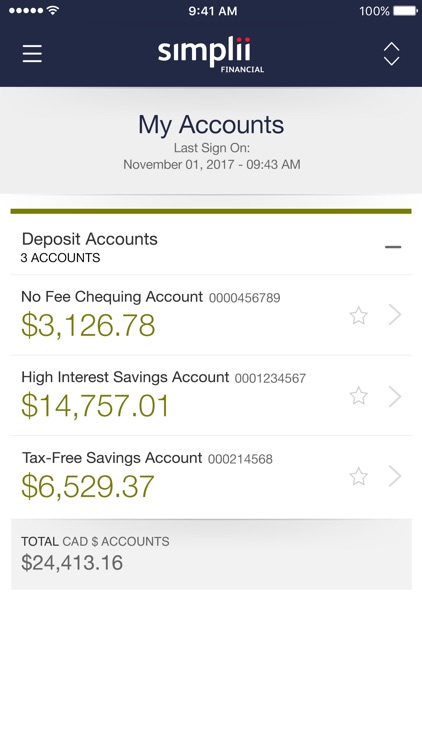Screenshot of a banking app interface, displaying detailed information and UI elements at the top, middle, and bottom parts of the screen. 

At the top, there are several status indicators: white circles, a white Wi-Fi symbol, the time displayed as 9:41 AM, and a battery indicator at 100%. Below these, a navy banner with white lines prominently features the logo "Simplii Financial," where the double 'i's are accented with small pinkish-red dots. 

Underneath the banner, there are two arrows in white, one pointing up and one pointing down. Further down, there’s a gray box with "My Accounts" written in navy text, followed by the sign-in time noted as "Last sign on, November 01, 2017, 9:43 AM" in gray.

Moving down, a green line separates the sections. Below it, in black text, it reads "Deposit Accounts, 3 accounts", accompanied by a minus sign for collapse/expand function. Listed beneath are three accounts:

1. **No Fee Checking Account**
   - Account number (omitted for privacy)
   - Balance: $3,126.78 displayed in a greenish-gold font
   - Accompanied by a gray star and a gray arrow

2. **High Interest Savings Account**
   - Account number (omitted for privacy)
   - Balance: $14,757.01
   - Accompanied by a gray star and a drop-down arrow 

3. **Tax-Free Savings Account**
   - Account number (omitted for privacy)
   - Balance: $6,529.37
   - Accompanied by a gray star and a drop-down arrow 

At the bottom, there is a summary labeled "Total CAD Accounts" showing a cumulative balance of $24,413.16.